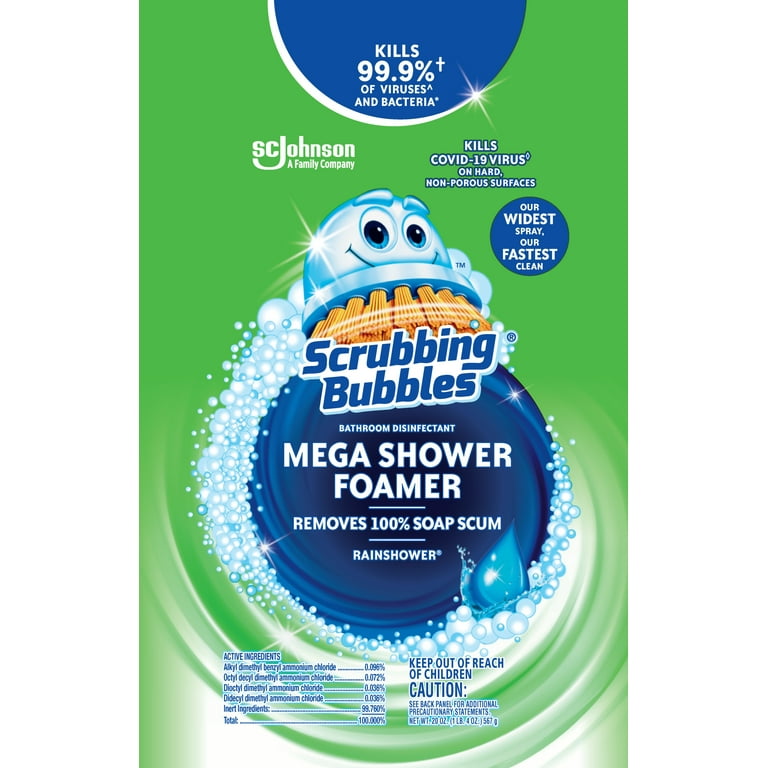The image is of a Scrubbing Bubbles cleaning product box. The background is primarily green towards the bottom, transitioning into a white half-circle in the center. At the top, a blue half-oval with a white starburst lines the edge. Inside the blue half-oval, in capitalized, centered white text, it says "Kills 99.9% of viruses* and bacteria," with the "99.9%" prominently displayed.

Below this blue section, "SC Johnson" is written in larger white text, with "A family company" in smaller font beneath it. To the right, centered white letters on a blue-lined background say "Kills COVID-19 virus," followed by "on non-porous surfaces" in smaller text.

One of the standout features is the Scrubbing Bubbles mascot— a smiling brush with blue and white bristles arranged like a dome. The brush has googly eyes, blue eyebrows, and a band transitioning from white to blue. Around the mascot are blue and white bubbles, cascading downwards and encircling a textured navy blue oval with a water droplet at the bottom right.

In large text beneath the mascot, it says "Scrubbing Bubbles®" and "Bathroom Disinfectant," followed by "Mega Shower Foamer" and "Removes 100% Soap Scum." The text sizes vary, with "Mega Shower Foamer" being the largest. "Rain Shower" is written beneath, alongside a small ® symbol.

To the left of the product information, a block of text labeled "Active Ingredients" lists various components, each with corresponding percentages in a right-aligned format. To the right, in a smaller font, a cautionary note reads "Keep out of reach of children" followed by a "Caution" notice, urging readers to "See back panel" for more details.

Overall, the box highlights the product’s ability to kill 99.9% of germs, including COVID-19, and emphasizes its effective cleaning properties with large, bold text and numerous detailed design elements.